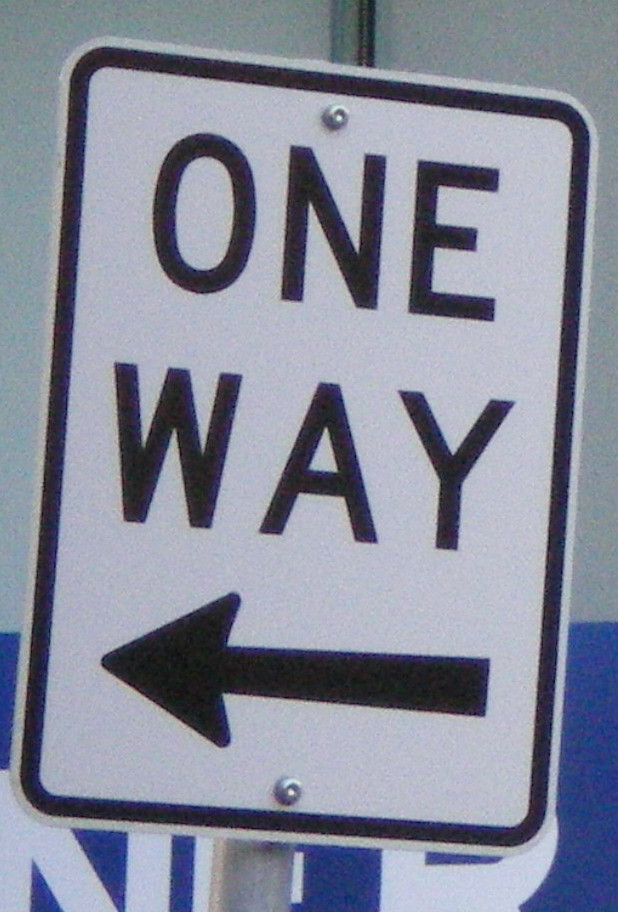This photograph features a close-up view of a "One Way" traffic sign. The sign is white with a black border and displays black text and an arrow pointing to the left. It is securely attached to a gray metal pole with two visible silver bolts; one bolt is positioned at the bottom center, and the other at the top center of the sign. Just above the "One Way" sign, part of the pole extends out of the frame, suggesting the possible presence of another sign not captured in this image. The background of the photograph shows a partial view of a white area at the top and a blue section with indistinct large white block letters at the bottom. The image itself is somewhat blurry and grainy, perhaps due to overexposure or age, giving it a textured appearance. The camera is positioned directly in front of the sign, providing a nearly perpendicular and very close perspective.